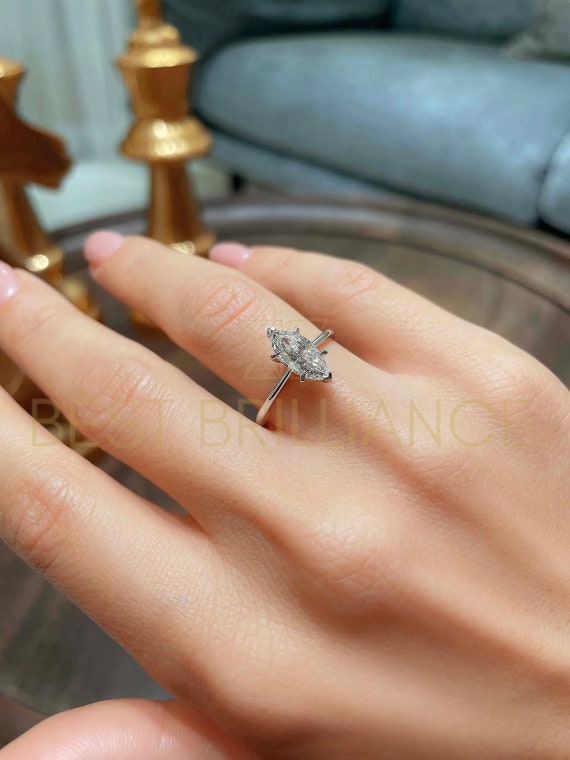In the image, there's a close-up of a woman's right hand with her fingers elegantly poised above a glass coffee table. Her nails appear well-manicured, showcasing her attention to detail. She's wearing a dainty, teardrop-shaped solitaire engagement ring on her ring finger. The ring features a high-quality, white diamond set on a thin silver band, reflecting her refined taste. Over her hand is a semi-transparent watermark text reading "Best Brilliance." The coffee table below her hand exhibits a couple of slightly out-of-focus golden candlesticks in the top left corner. In the top right corner, there's a hint of a bluish-green sofa, also blurred, suggesting a cozy, stylish setting.